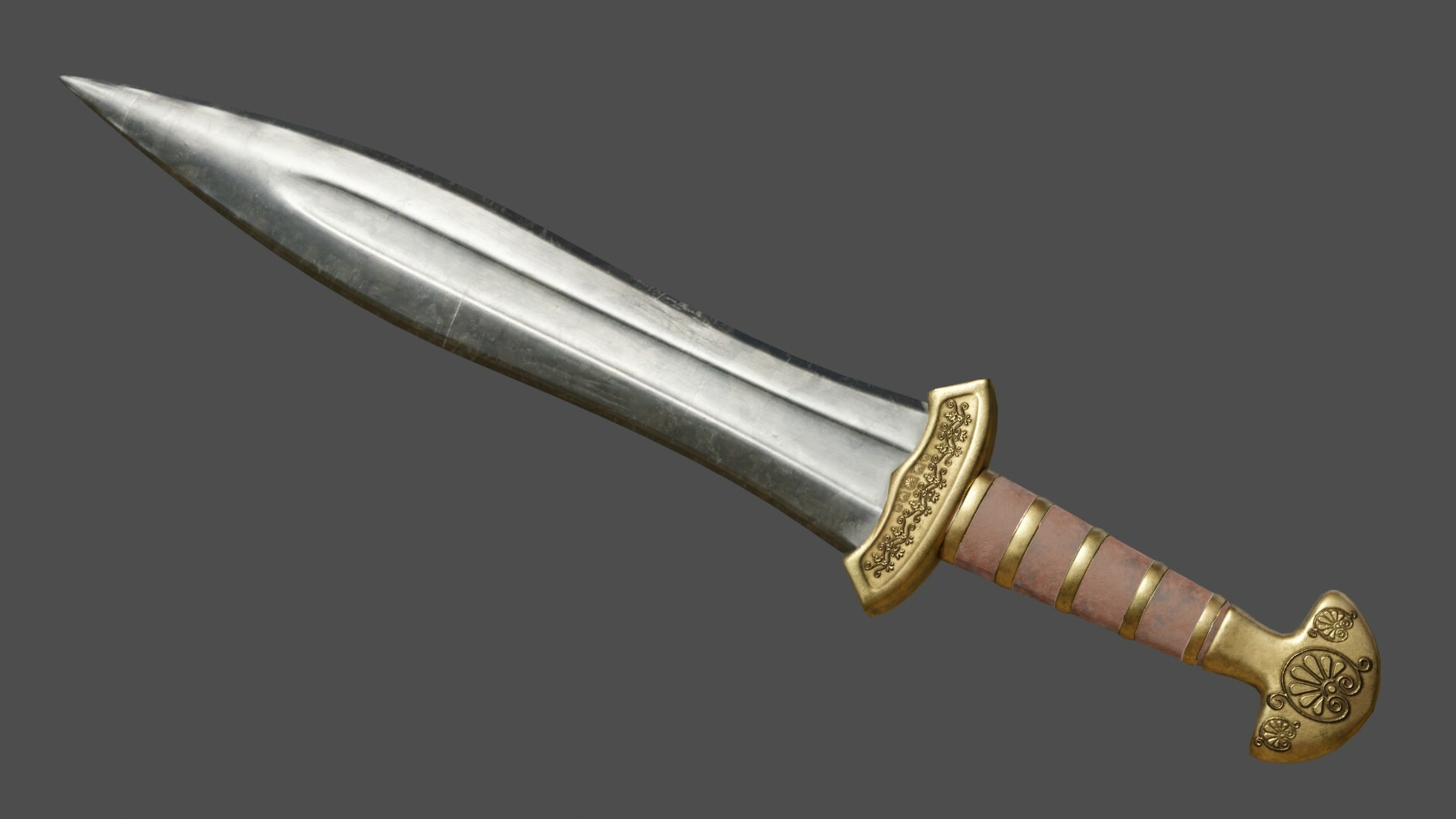The image showcases an antique dagger prominently displayed against a dark gray horizontal background. The dagger features a silver blade with a distinct ridge along its side, exhibiting signs of wear and tear. The blade tapers to a sharp point. The handle is brass-colored and wrapped with brown leather strips, possibly to enhance grip. Near the base of the blade, there is an ornate gold or bronze hilt, designed to protect the hand, with detailed engravings. The end of the handle boasts a semi-circular design with intricate carvings reminiscent of shells, adding to its decorative appeal.